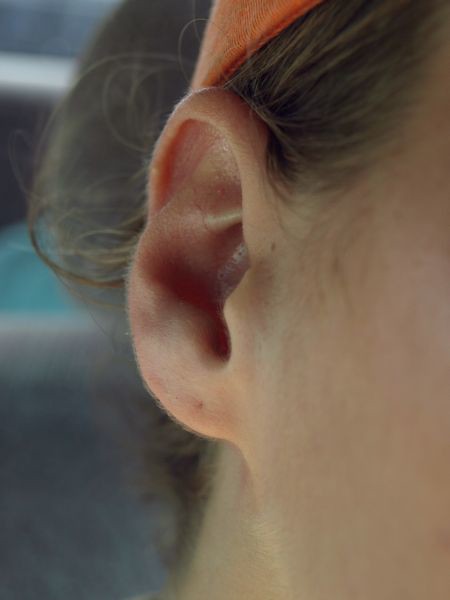The close-up photograph showcases the right ear of a young Caucasian woman with light brown hair, which is tied back into a bun by an orange fabric headband. The focal point of the image is her ear, which appears smaller than average, with a particularly diminutive earlobe and an upper part that seems to sink slightly into her head. The ear's skin is notably thin and veiny, suggesting an unusual medical condition. The clarity of the image, enhanced by natural light, also reveals a piercing on the lower part of her earlobe, though it lacks an earring. The smoothness of her visible cheek and neck further hints at a younger age, but no facial features like eyes, nose, or mouth are discernible. The setting is bright, highlighting the details of the woman's ear and the orange headband.